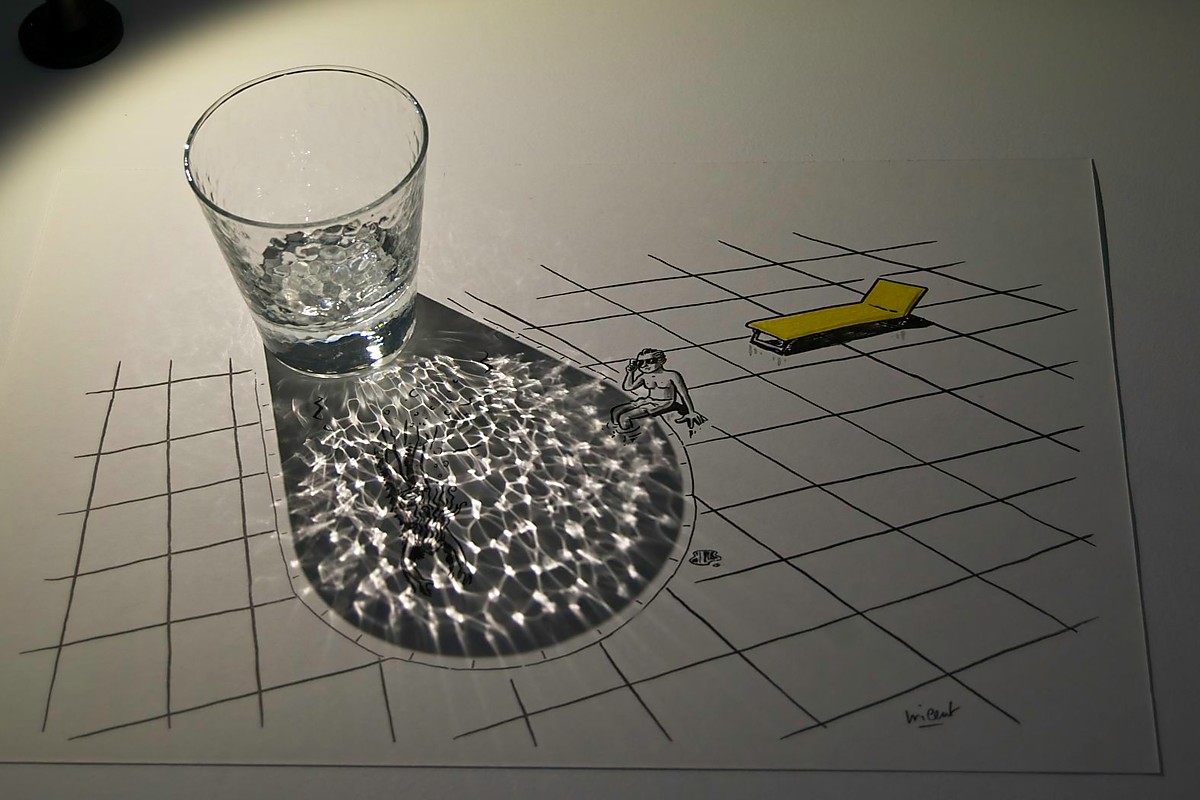In this imaginative and detailed drawing, a clear textured glass placed on a sheet of paper creates a sunlit pattern resembling the shimmering water of a swimming pool. The artist has cleverly accentuated this effect by drawing a border around the light reflection and adding a cartoon-like pool scene. There's a man in sunglasses sitting on the pool's edge, dipping his feet into the 'water'. Additionally, a person is illustrated swimming beneath the water's surface. The poolside features a yellow reclining chair, adding a splash of color to the predominantly black-and-white sketch. The background of the artwork includes a diagonal grid pattern, enhancing the aesthetic appeal. The drawing is signed at the bottom corners, though the signature is illegible. A small black dot is noticeable in a darkened upper left corner of the paper, contributing to the intricate details of this creative piece.